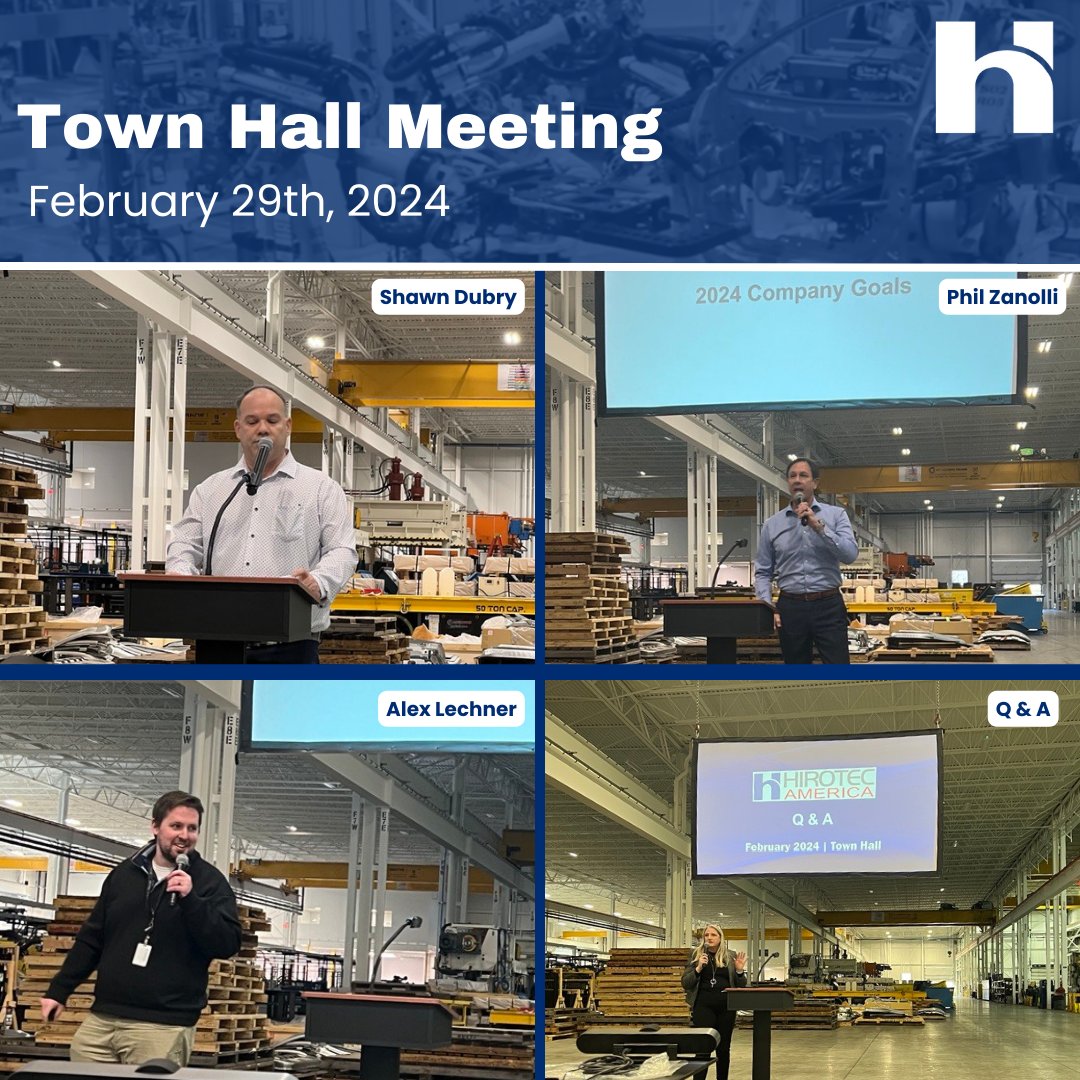This image portrays an announcement for a Town Hall Meeting held by Herotech America on February 29, 2024. The top section of the image is marked by bold, white text on a blue background, stating "Town Hall Meeting," with the date directly below. The right side prominently displays Herotech's logo, featuring a unique stylized combination of a lowercase and uppercase "H."

The image is divided into a 2x2 grid of webcam screenshots, with each square highlighting a different participant against the backdrop of a warehouse filled with wooden pallets and high industrial ceilings:

1. **Top Left**: Sean Dobry stands at a podium, appearing engaged in his speech.
2. **Top Right**: Phil Zanoli, also at a podium and using a microphone, is positioned under a large projector screen.
3. **Bottom Left**: Alex Lechner, wearing a black jacket, is caught in a moment of laughter while holding a microphone.
4. **Bottom Right**: A blonde woman, part of the Q&A session, stands beneath another projector screen.

Each participant's name is labeled just above their respective images, emphasizing their roles in what appears to be a lively, well-organized town hall event.